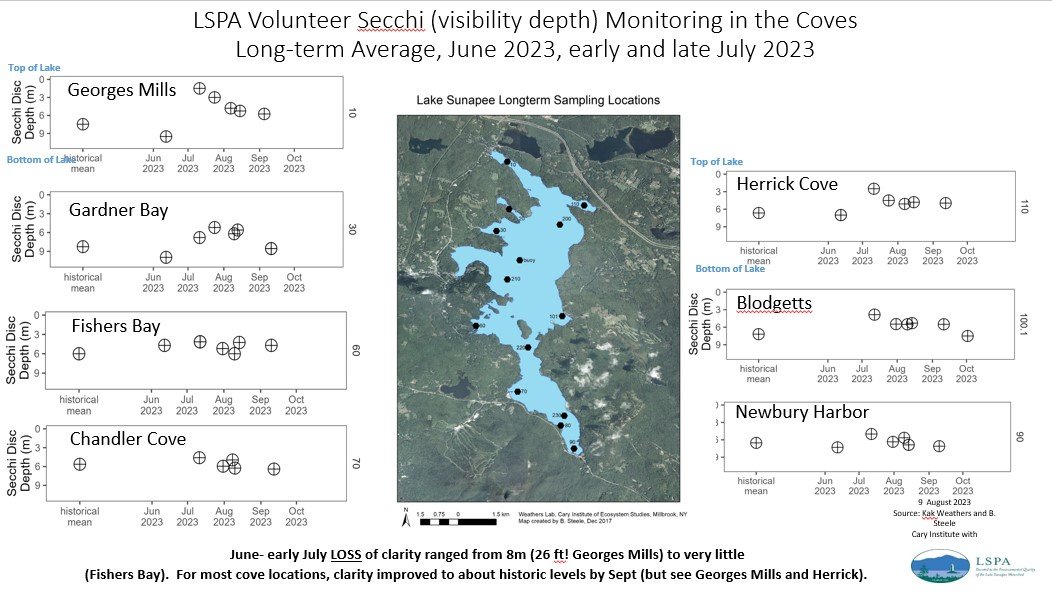The image is a detailed diagram featuring a central map with a green landmass and a blue water body, likely representing Lake Sunapee. The map has numerous black dots indicating various sampling locations. At the top, the caption reads "LSPA Volunteer Sechi," with a note in parentheses stating "Visibility Depth Monitoring in the Coves, Long-Term Average, June 2023, Early and Late July 2023." Below this, an overlay text specifies "Lake Sunapee Long-Term Sampling Locations."

Flanking the central map, there are thin black rectangular keys on the left and right sides, containing circles with crosses inside them and labeled with different sampling site names and corresponding data points. The left side lists places such as Georges Mills, Gardner Bay, Fishers Bay, and Chandler Cove, while the right side includes Herrick Cove, Blodgetts, and Newbury Harbor.

In the bottom section of the diagram, additional text details the study's findings: "June to early July loss of clarity ranged from 8 meters (26 feet) at Georges Mills to very little at Fishers Bay. For most cove locations, clarity improved to about historic levels by September, but see Georges Mills and Herrick." A logo featuring an oval with mountain terrain and the acronym "LSPA" is positioned at the lower right corner. The background of the entire diagram is plain white, ensuring the information is clearly visible.